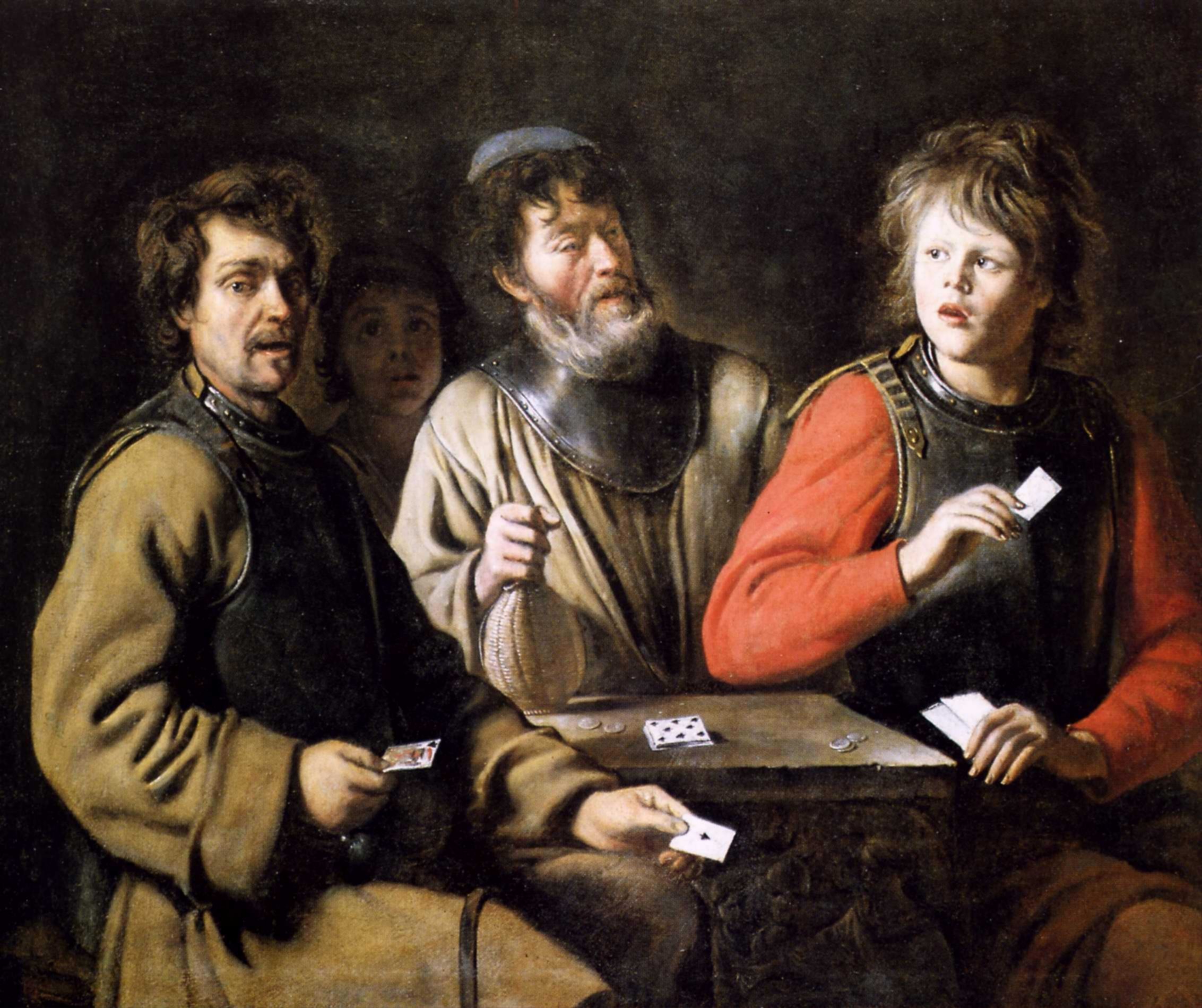This painting depicts four individuals, three of whom are engrossed in a card game while the fourth stands in the background, looking concerned. The setting is characterized by a small central table with playing cards and coins, indicating a gambling scene.

On the left side sits a man with wavy brown hair, a mustache, and pale skin, clad in a black vest over a green robe or tunic. He holds two playing cards, a king and an ace, with a serious demeanor. Next to him, seated behind the table, is an older man with dark curly hair partially covered by a dark grayish-blue cap. He has a tan robe, a gray beard, and a black collar, holding a canteen, possibly of liquor. His attire includes what appears to be leather or metal chest armor.

To the right sits a youthful-looking figure, despite their adult stature. This individual has wavy brown hair and a childlike face with no facial hair, dressed in a red tunic with a black vest. The fourth person, in the background, has dark brown hair, wide-open eyes, and a downward-turned mouth, conveying a scared or anxious expression as they gaze at the man in the green robe.

The entire ensemble is painted using a palette of black, white, gray, red, green, tan, taupe, brown, and blue. The backdrop features varying shades of dark browns, which adds depth and mood to the scene. The painting's style and the characters' attire suggest an attempt at a historical or allegorical representation, though its exact period remains ambiguous. There is no text included in the artwork.